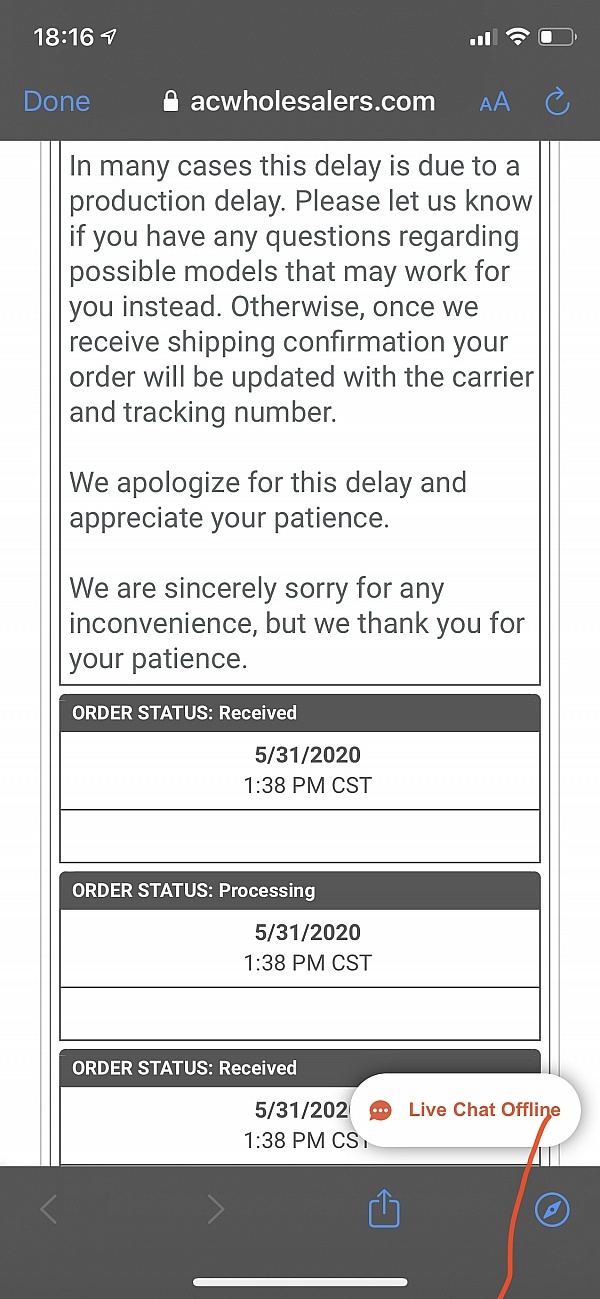This is a detailed caption for the screenshot you described:

---

A screenshot of a smartphone displaying a customer service message from ACWholesalers.com. The top left corner shows the time "18:16" along with the word "Done" just below it. In the center at the top, there is a padlock icon indicating a secure connection, the website URL "ACWholesalers.com," and three vertical bars representing a full data signal. Next to these, Wi-Fi and battery symbols are shown, with the battery being about one-fourth charged. 

On the right side, there are two blue-letter "A" icons for text sizes, followed by a blue refresh symbol. The message below reads: "In many cases, this delay is due to a production delay. Please let us know if you have any questions regarding possible models that may work for you instead. Otherwise, once we receive shipping confirmation, your order will be updated with the carrier and tracking number. We apologize for this delay and appreciate your patience. We are sincerely sorry for any inconvenience, but we thank you for your patience."

Further down, order status updates are listed:
- "Order status received: 05/31/2021 1:38 PM CST."
- "Order status processing: 05/31/2021 1:38 PM CST."
- "Order status received: 05/31/2022 1:38 PM CST."

The notification indicates that live chat is currently offline, with a red line drawn through the "Offline chat" section. At the bottom, navigation icons include a left arrow, a right arrow, an upload symbol, a compass icon, and a white dash in the center, likely part of the phone's interface.

---